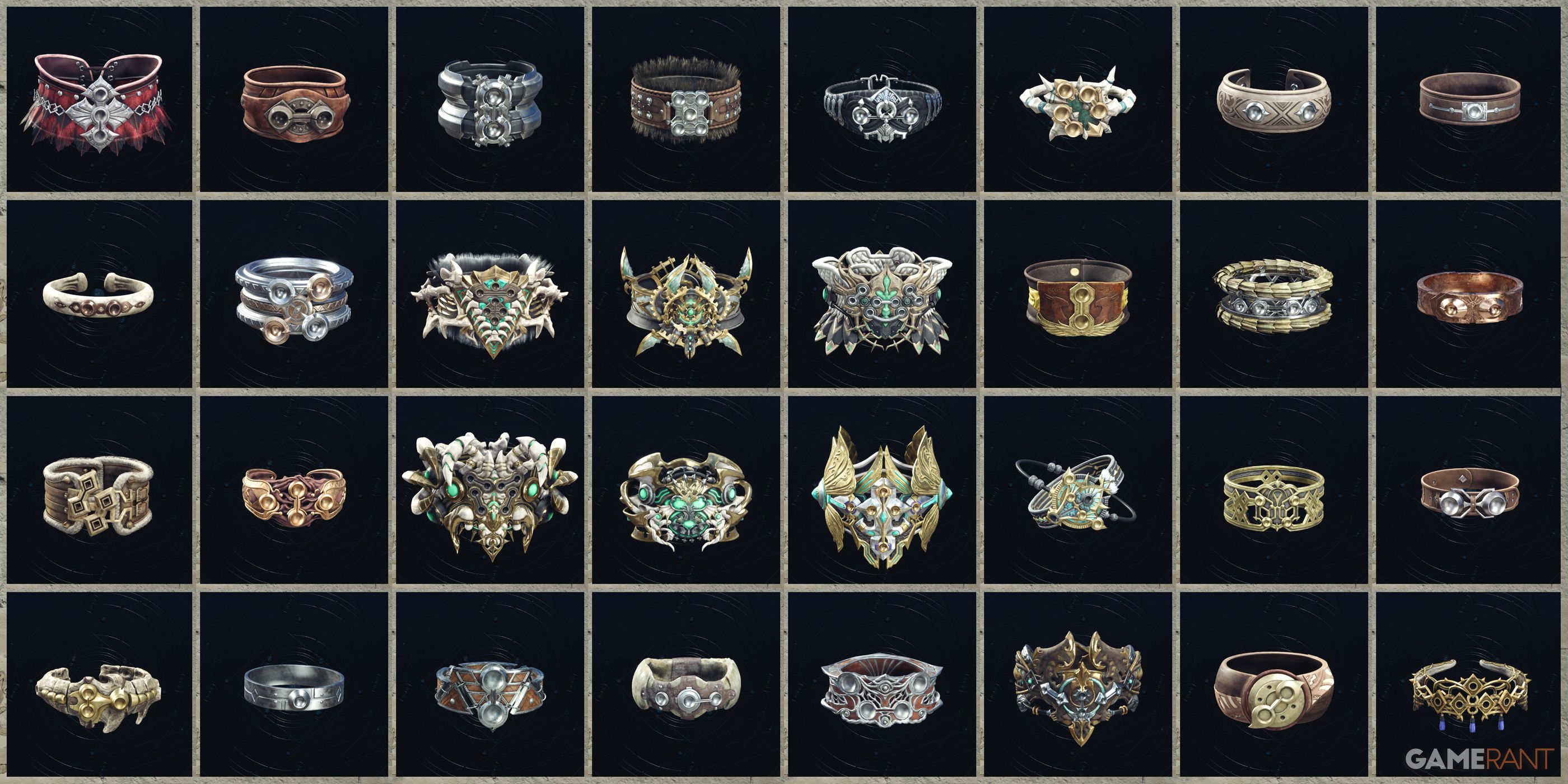This image showcases a collection of intricately designed, fantasy-style rings arranged in a grid format. The display features four rows and eight columns, totaling 32 rings, each housed in its own black cubby hole. The rings vary in shape, size, and design, with some adorned with spikes, jewels, and ornate golden trims, while others feature more subdued metal finishes. The colors of the rings range from vibrant reds and blues to golds, bronzes, silvers, and whites. Some rings exhibit abstract designs or face motifs, adding to their otherworldly charm. The bottom right corner of the image has the words "GAME RANT" in an all-caps, fine font, with "GAME" in white and "RANT" in orange.